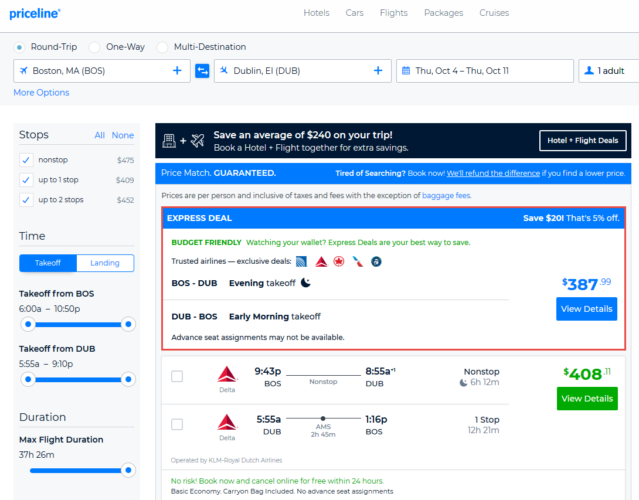A screenshot from the Priceline website details various booking options available for a trip from Boston, Massachusetts to Dublin, Ireland. The top navigation bar features clickable sections for hotels, cars, flights, packages, and cruises. Below these options, users can select their trip type with choices like round-trip, one-way, or multi-destination. 

In this particular search, the trip is scheduled from October 4th to October 11th, with one adult traveler specified, although additional travelers may be included beyond what's visible in the cut-off portion of the page.

The focal point of the image highlights an "Express Deal" section, which is outlined with a prominent red rectangle. This promotion advertises a $20 discount, equivalent to 5% off, emphasizing budget-friendly travel. The text in this section encourages travelers to consider "Express Deals" for the best savings, with mentions of trusted airlines offering exclusive deals. Specifically, the flight from Boston to Dublin departs in the evening, and the return flight from Dublin to Boston takes off early in the morning. The total cost for this deal is $387.99, and there is an option to view more details.